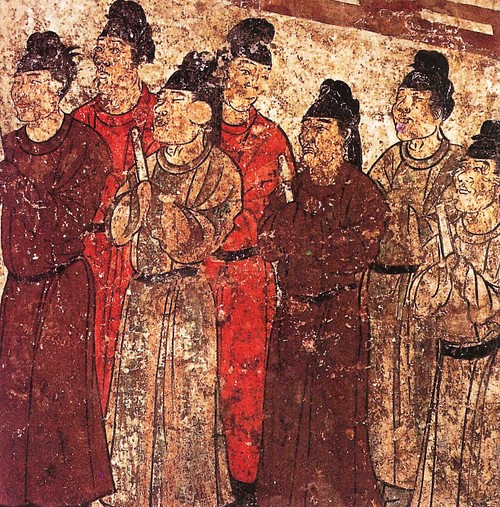This artwork appears to be an ancient East Asian illustration, possibly Japanese or Chinese, dating back several centuries. It depicts six men, all with distinctively styled hair in topknots, suggesting they may be monks or scholars. They stand solemnly in a row against a plain, white splotchy background. The men are dressed in robes of varying colors—two in vibrant red and others in faded shades of brown, cream, and maroon, indicative of aged ink. Each holds an object in their hands; three appear to be holding candles or possibly scrolls, adding to the solemn, contemplative nature of their gathering. Their faces bear quizzical expressions, enhancing the sense of mystery and depth in the scene.